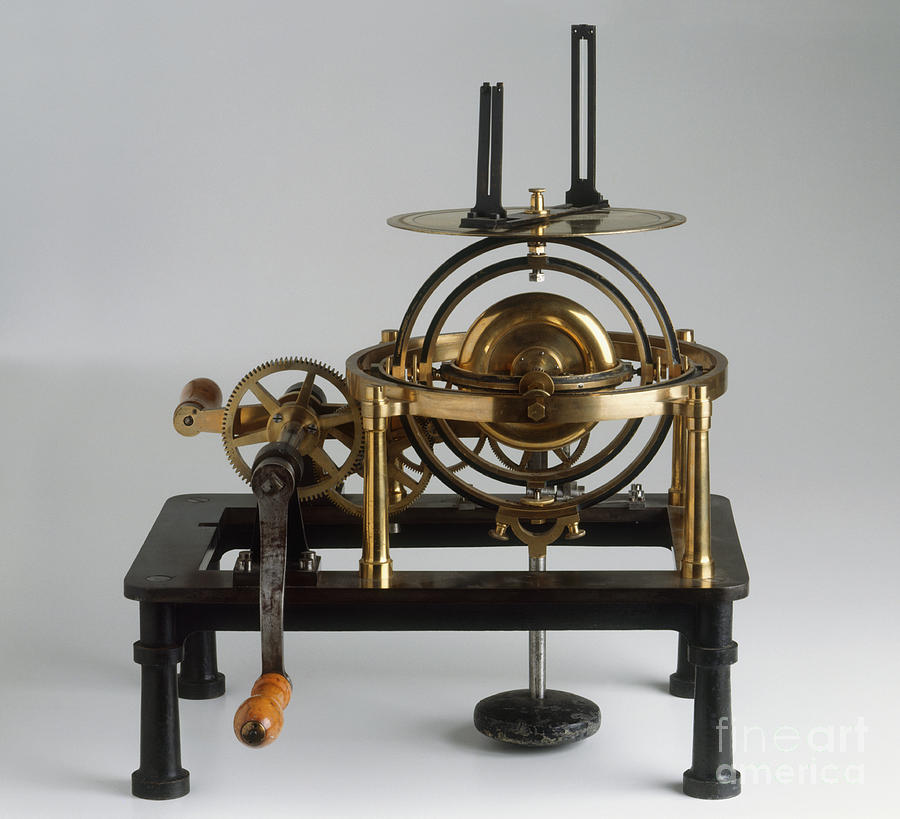The image showcases a detailed model of an old machine set against a plain white background and white table. The machine prominently features a black metallic base resembling a rectangular coffee table with four legs. At the left of the base is a metal handle with a wooden knob, which connects to a shiny gold gear, suggesting it could be cranked by hand. The central portion of the machine is dominated by interconnected bronze and gold-colored metal circles and cogs, forming what looks like a mechanical globe or an intricate gear system. Extending from this central arrangement is a flat circular piece of gold metal, topped with two protruding black poles. The overall design appears to be a historical piece of machinery, hinting at its possible upgrades over time. Despite its enigmatic purpose, the craftsmanship showcases a blend of black and bronze metals with a focus on gears and rotational components.